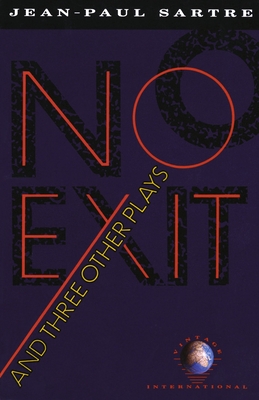The image is of a book cover with a deep purple background. At the very top, there is a black strip with the author’s name, "Jean-Paul Sartre," written in bold, wide white letters. The title, "No Exit," is prominently displayed in large, thin red text, each letter outlined with a speckled black drop shadow that gives it a striking effect. Notably, the diagonal line of the 'X' extends down to the bottom left corner, forming a base for the subtitle, "and Three Other Plays," which is written in yellow text, slanting upward towards the 'O' in "No." Additionally, there is a secondary offset shadow effect on the 'O' of "No," adding depth to the design. The bottom right corner of the cover features a globe emblem with the words "Vintage" arced over it and "International" in a straight line beneath, identifying the publisher. This detailed and theatrical cover design effectively highlights the dramatic content of Sartre's plays.